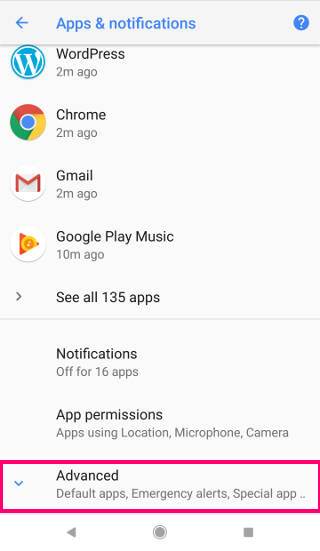The image is a detailed Android mobile screenshot, characterized by familiar navigation icons at the bottom—a leftward-pointing arrow, a circle, and a square. At the top of the screen, within a blue banner that reads "Apps & notifications," a blue left-pointing arrow is prominently displayed alongside a blue circle containing a white question mark, suggesting contextual help or information.

The screenshot lists several apps with recent activity:
1. The first app icon is a medium blue circle featuring a stylized white "W" representing WordPress, with the text "2 minutes ago" indicating recent use.
2. Below it is the Chrome browser icon, a circle segmented into red, yellow, and green with a blue dot in the center, also showing activity "2 minutes ago."
3. The Gmail icon follows, displaying a white envelope with red accents, likewise marked with "Gmail 2 minutes ago."
4. Farther down, there's the Google Play Music icon, a red play button with a small yellow clock overlay, showing activity "10 minutes ago."

Further down, the screen displays the option "See all 135 apps" and indicates that "Notifications off for 16 apps." It lists additional settings such as "App permissions," "Apps using location," "Microphone," and "Camera."

A red-highlighted section reading "Advanced" captures attention with sub-options including "Default apps," "Emergency alerts," and a partially visible "Special app…" suggesting more hidden settings.

The overall screenshot illustrates navigational steps within the "Apps & notifications" settings menu on an Android device, offering access to various app-specific configurations and permissions.